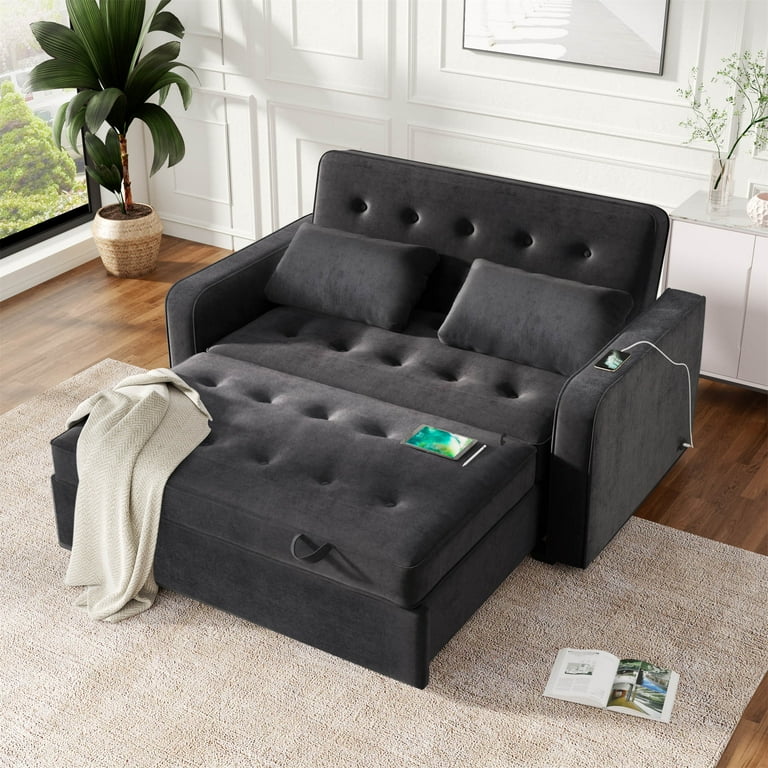The photograph captures the interior of a well-lit room with a white background, featuring a dark gray, contemporary sectional sofa. This sofa includes an extended ottoman that seamlessly integrates with the main seating, providing ample space to stretch out comfortably. Adorning the couch are two matching gray pillows and a light blanket draped on one side. A tablet displaying blue and green hues rests on the ottoman, while a phone, charging via a cord that runs to a concealed USB port, sits on the armrest. 

The floor showcases beautiful hardwood with a partly covering soft white throw rug. Scattered around are a few elements that add a lived-in feel: an open book on the sofa, a magazine on the rug, and a lightweight jacket, or blanket, casually left on the side. The room basks in natural sunlight streaming through a nearby window, which offers a view of a road lined with green trees. The setting is completed by the presence of a healthy potted plant with large leaves in the background, enhancing the room's cozy and inviting atmosphere.